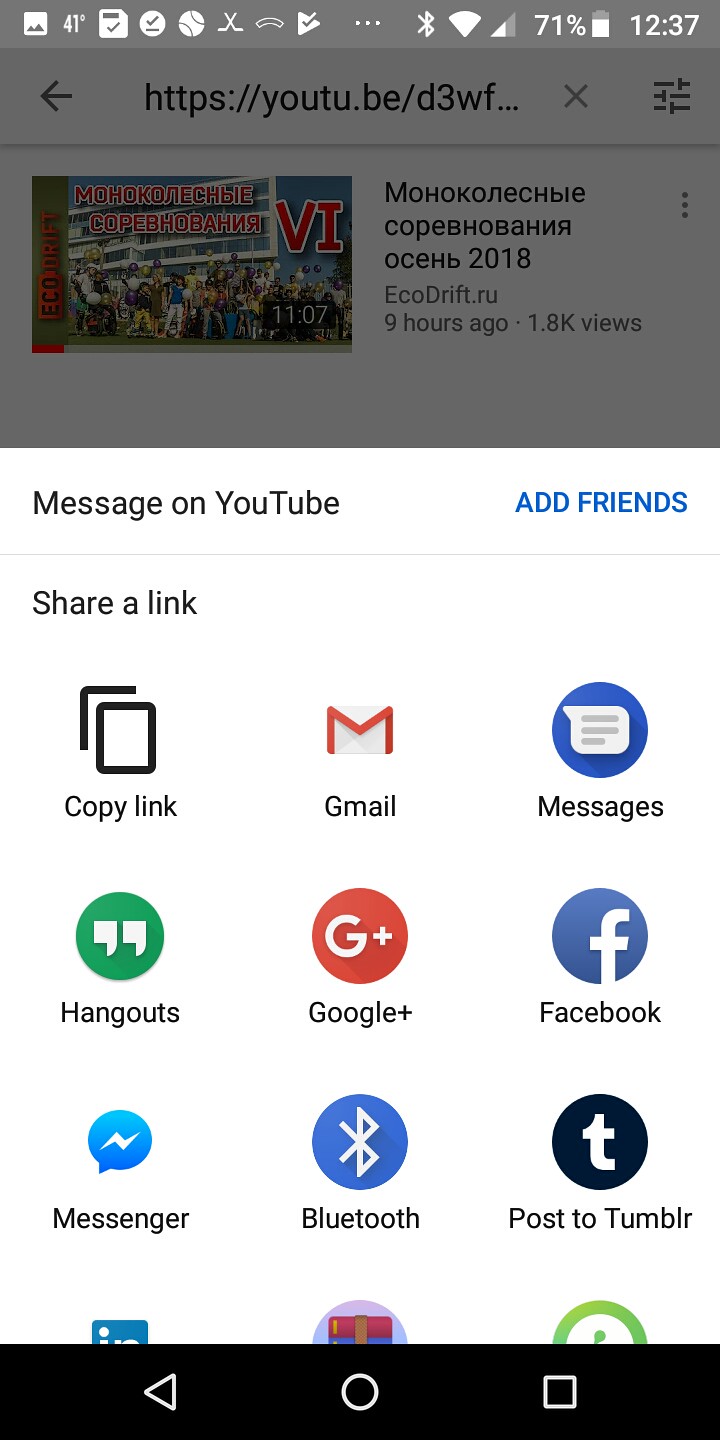This photo captures the screen of a smartphone, displaying various app icons and notifications. At the top, there is a gray rectangular notification bar in landscape orientation featuring several icons: a message notification, a picture, a file download, an update alert, a baseball, a Google update, and a Bluetooth icon. The battery level is at 71%, and the time displayed is 12:37.

Below the notification bar, there is a YouTube video clip in a foreign language that is 11 minutes long. The video is framed within a white border that is in portrait orientation. Beneath the video, in black text, it mentions, "Message on YouTube," with an option to the right in blue letters reading, "Add friends." The section below provides options for sharing a link, labeled "Share a Link," which offers various platforms for sharing.

The sharing options are organized into rows:
- The first row includes "Copy link," "Gmail," and "Messages."
- The second row features "Hangouts," "Google Plus," and "Facebook."
- The third row includes "Messenger," "Bluetooth," and "Post to Tumblr."

Below the third row, only half of a link icon is visible, along with two partially cut-off icons that are not easily recognizable. The overall screen suggests that the person is in the process of sharing a YouTube video across different platforms.